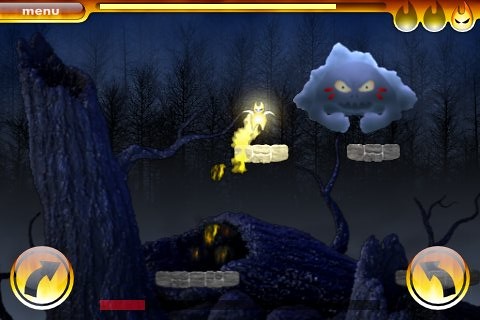This screen capture from a video game depicts a dramatic nocturnal scene. Dominating the image are two yellow circular icons with smaller black concentric circles within, positioned near the top corners of the screen with curved black arrows pointing inward towards the horizontal center. The background reveals a dark and moody landscape with the silhouette of a cliff and trees set against a pitch-black sky. Central to the image is a yellow figure, potentially an animal or object, with a large green pea-like shape beneath it. To the upper right of this figure, a lighter gray cloud takes on an anthropomorphic form, featuring a menacing expression with furrowed yellow eyes, red cheek marks, and clenched fists held forward. Below this cloud figure lies a four-brick stone wall. Additionally, the upper right corner of the screen displays several teardrop-shaped yellow symbols with slanted black eyes, enhancing the game's eerie atmosphere.